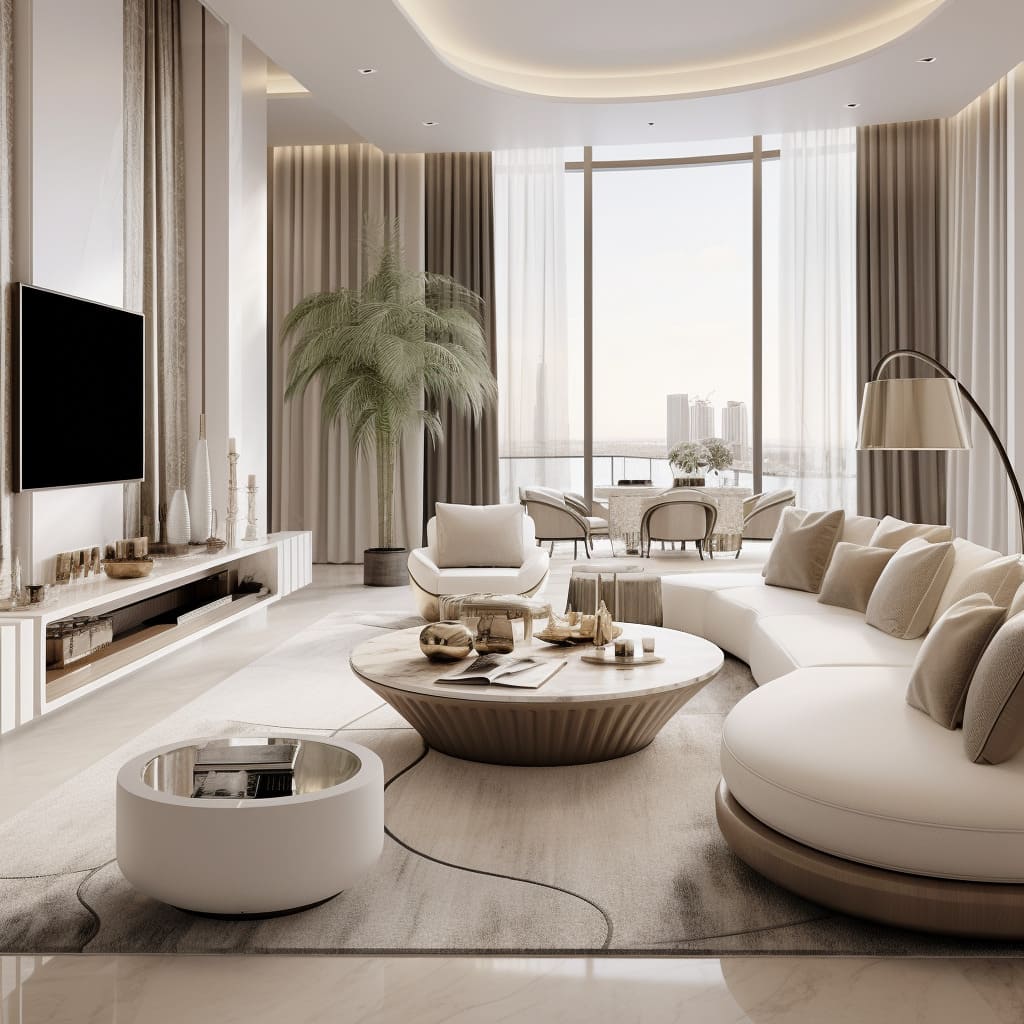The image captures a high-end, monochrome-neutral living room inside a luxury high-rise apartment, bathed in a mix of natural and artificial light. Dominating the central area is a large picture window, offering a view of distant skyscrapers. The living room features a sleek, cream-colored sectional couch adorned with square light brown pillows. Adjacent to the couch is a round coffee table holding some glasses and magazines, alongside smaller circular end tables. Opposite the couch, a television is mounted on the wall above a white entertainment center decorated with various items. The left wall is a crisp white, contrasting with floor-to-ceiling windows on the right side, framed by tall, brown and ivory curtains. Grounding the space, the floor showcases light brown wood-patterned tiles. In the dining area, a round table surrounded by cushioned beige chairs sits partially up the picture, framed by the upscale interior’s sophistication.